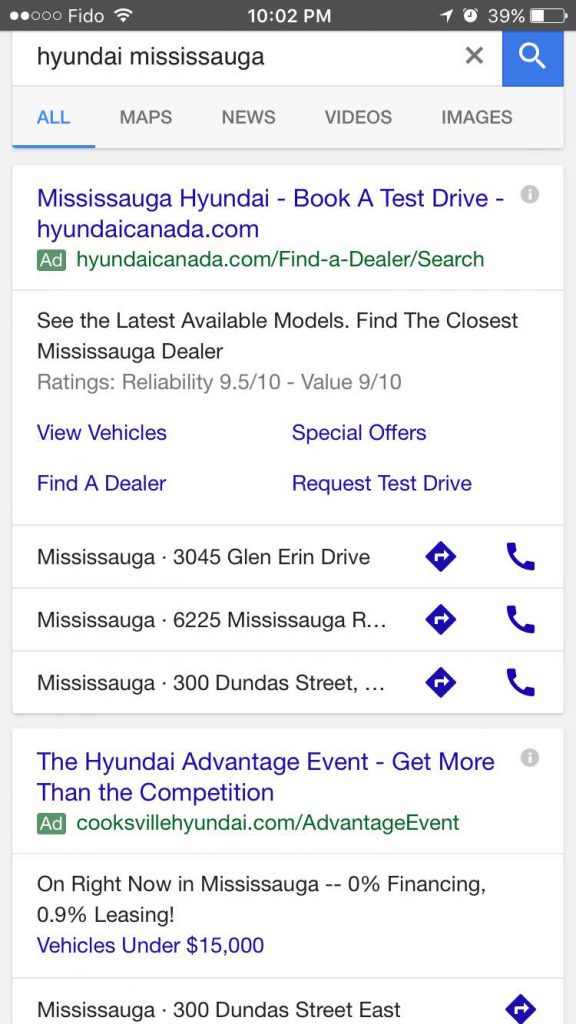**Detailed Screenshot Description:**

This screenshot captures the display of a smartphone with visible time, network, and battery indicators. At the top, a black banner shows "Fido" in white font, followed by standard network icons, the time "10:02 PM," a send icon, and a battery icon indicating 39% charge.

Below this, the screen transitions to a white background highlighting a search result for "Hyundai Mississauga." An 'X' and a microscope icon over a blue background are located just below the search term. Below these icons, several tabs list options such as "All," "Maps," "News," "Videos," and "Images."

The first content block underneath these tabs is an advertisement for Mississauga Hyundai. The ad, labeled as such, reads "Mississauga Hyundai - Book a test drive" with a link to "HyundaiCanada.com" in blue text. Below this, on a white background, there's a green square labeled "ad" next to "HyundaiCanada.com/find-a-dealer/search."

This is followed by promotional text in black declaring, "See the latest available models, find the closest Mississauga dealer," with ratings for reliability (9.5/10) and value (9/10) noted in gray. Blue hyperlinks offer actions including "View vehicles," "Special offers," "Find a dealer," and "Request a test drive."

Further down, the screen lists three Hyundai dealership locations in Mississauga:
1. 3045 Glen Erin Drive, accompanied by an arrow and phone icon,
2. 6225 Mississauga Road,
3. 300 Dundas Street.

Beneath these details, another ad proclaims "The Hyundai Advantage Event - Get more than the competition" in blue. This is followed by a green "ad" square linked to "CooksvilleHyundai.com/advantage-event."

The final section touts the current offers, stating "On right now in Mississauga - 0% financing, 0.9% leasing, vehicles under $15,000," along with the location "300 Dundas Street East" marked with an arrow, indicating another dealership or event spot in Mississauga.